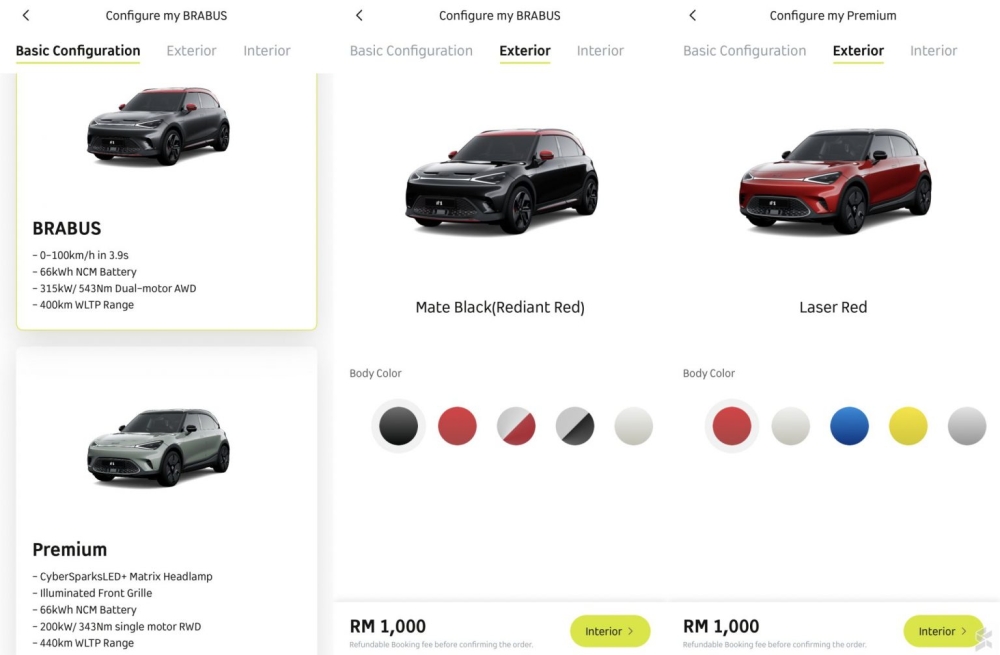This detailed caption describes multiple stages of a car customization process showcased on a website:

"The image series captures different stages of a car customization process on a website, evidently prior to the purchase of a vehicle. The first image displays the 'Configure my Brabus' section, highlighting the basic configuration options. Notable features include a performance specification of 0-100 km/h acceleration in 3.9 seconds, a 66 kWh NCM battery, a 315 kW power delivery, dimensions of 5x3 NM, dual motor AWD, and a 400 km WLTP range. Additional premium options like the Cyberspark sled, Matrix headlamp, and an illuminated front grille are visible. For a different configuration, there's a 66 kWh battery paired with a 200 kW single motor, offering a 440 km WLTP range.

The second image transitions to the 'Exterior' selection stage, showing the car with a matte black exterior and radiant red paint. The third image further elaborates on exterior customization, this time with a laser red color selected. Each stage offers a detailed look into configuring various features and color options for the car, providing a comprehensive customization experience for the user."